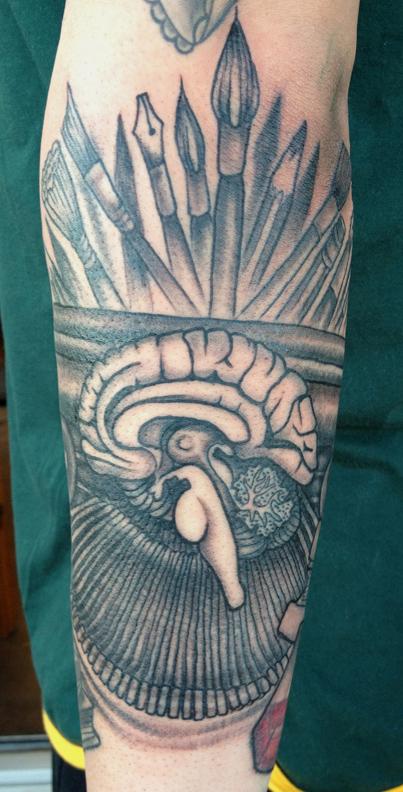The image showcases an intricate and detailed tattoo on a person's right arm, hanging down by their side. The tattoo spans a significant portion of the arm and is rich in artistic elements. At the top, various drawing instruments, including paintbrushes, pencils, and nib pens, are protruding upward, creating a dynamic and creative vibe. Below the artistic tools, a detailed and elaborate depiction of a brain is seamlessly integrated with surrounding imagery, making it appear complex and thought-provoking. The tattoo wraps around the arm like a band. Below this, there are what seem to be typewriter keys, adding to the artistic and possibly literary theme of the design. The person, light-skinned, is wearing a green top with yellow trim, accentuating the detailed and colorful nature of the tattoo, which includes shades of black, tan, yellow, dark green, and a hint of red. The photograph is a close-up, capturing both the tattoo and the attire clearly, yet the setting remains ambiguous as to whether it was taken indoors or outdoors.